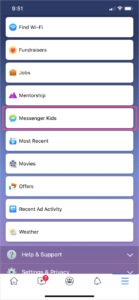A blurry screenshot of a mobile device screen displays an interface set against a gradient background transitioning from dark violet at the top to light purple at the bottom. The device's status bar at the top indicates the time as 9:51 AM on the left, with a signal strength at 50%, full Wi-Fi connectivity, and a nearly full horizontal battery icon on the right.

The screen showcases 10 rounded-corner rectangular bars, each with unique text and an accompanying icon, separated by small gaps that reveal the gradient background. The first bar reads "Find Wi-Fi" with a Wi-Fi symbol to its left. The second bar says "Fundraisers" and features a yellow icon with red details, though the specifics are unclear. The third bar is partially illegible but appears to start with "Jibo." The fourth bar, "Membership," includes a mountain icon to its left. Next, "Messenger Kids" displays the Facebook Messenger icon and is highlighted with a hot pink outline added by the user. Subsequent entries include vague or partially visible labels such as "most recent," "Mayhem" or "Mayless," "offers," "recent ad activity," and "weather."

Below these bars are two transparent accordion dropdown menus. The first dropdown menu, labeled "Help and Support," includes a question mark icon, while the second, "Settings and Privacy," features a cogwheel icon.

The bottom navigation bar of the app includes icons for home, video (with a red notification badge displaying the number 7), groups, notifications, and a three-line hamburger menu. The bottom central portion of the image has a dark blue outline, marking the end of the image.